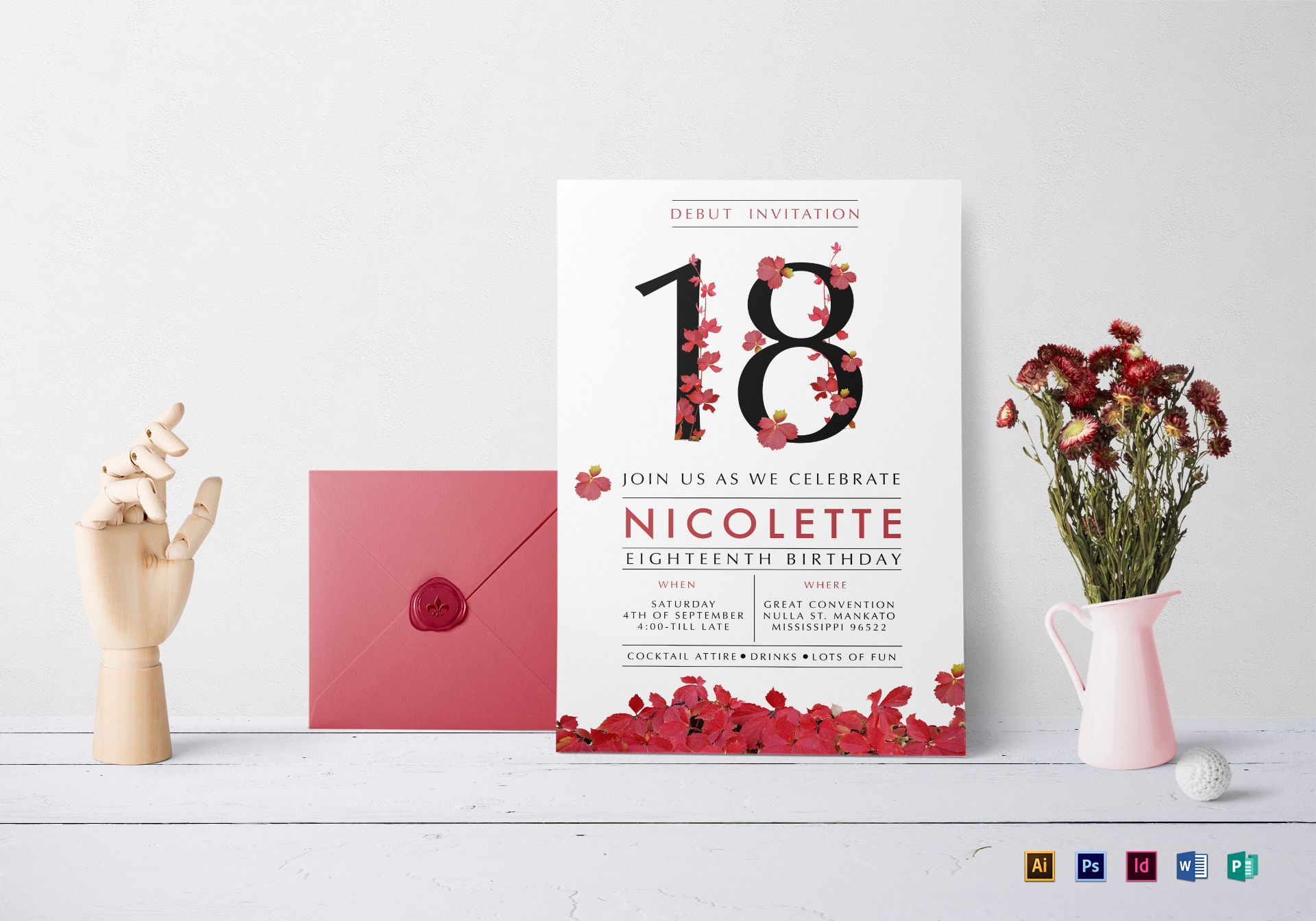The image is an advertisement for various computer programs, showcasing a styled birthday invitation for Nicolette's 18th birthday. The invitation is displayed standing on a flat surface resembling white wood paneling, with icons for Adobe Photoshop, Illustrator, InDesign, Microsoft Word, and Publisher in the bottom right corner, indicating the tools used to create it. 

The invitation features bold black numbers "18" adorned with pink flowers. The main text reads, "Debut invitation 18. Join us as we celebrate Nicolette's 18th birthday," followed by the event details: "When? Saturday, 4th of September, 4 till late. Where? Great Convention NOLA, St. Mankato, Mississippi, 96522. Cocktail attire. Drinks. Lots of fun." Below the text, there are scattered red rose petals.

To the left of the invitation is a red, wax-sealed envelope with a fleur-de-lis imprint, adding an elegant touch. Beside the envelope is a posable wooden mannequin hand, often used for drawing. On the right side, a pink pitcher serving as a vase holds reddish-pink flowers, and in front of it sits a decorative white ball. The entire arrangement is set against a stylish gray background, pulling together a refined and festive composition.